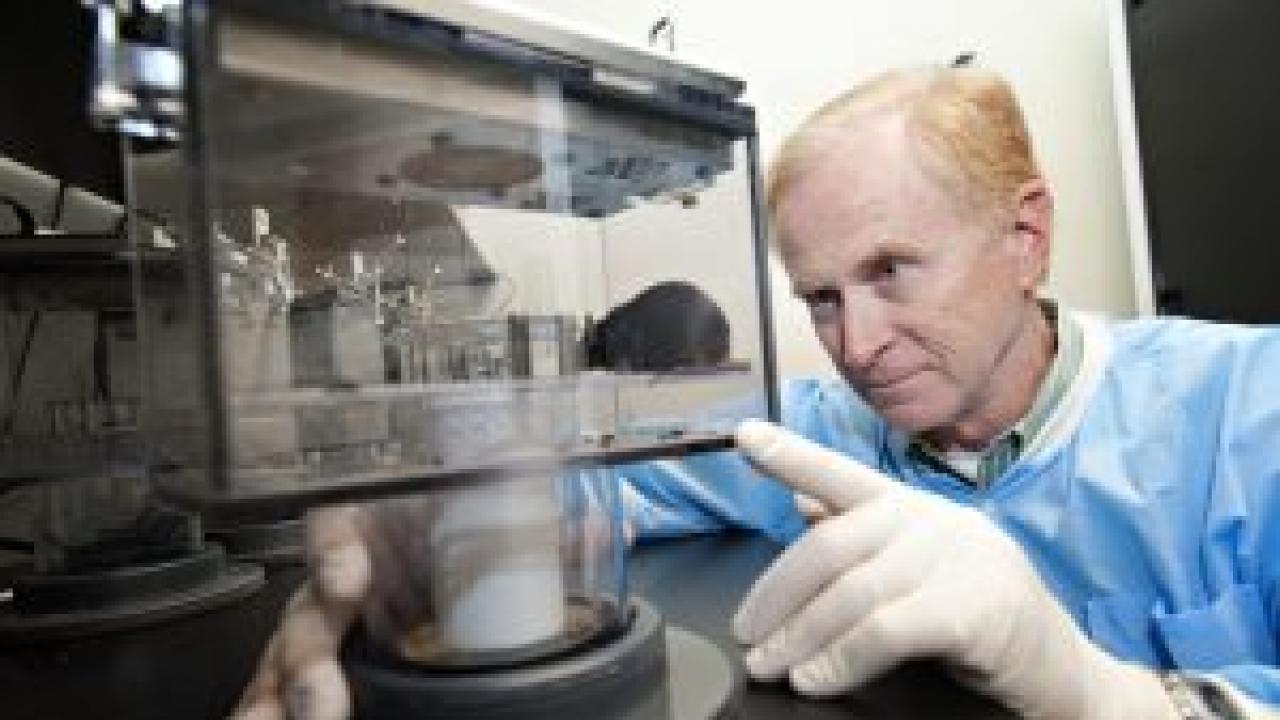The photograph features an older Caucasian male scientist, likely in his 50s, with light blonde or strawberry blonde hair and light facial features. He is dressed in a blue lab smock over a collared shirt, white gloves, and a wristwatch. Positioned on the right side of the image, the man is deeply focused on observing a glass cage or rectangular box with glass or plastic sides. Within the container, there appears to be a mouse, which the scientist is studying intently. The box has a cylindrical mechanism attached to it, possibly for experimental purposes. The scene is set in a laboratory environment, with various technical equipment present, suggesting that the scientist is conducting or observing an experiment. The photograph is somewhat blurred, emphasizing the intensity and concentration of the man's gaze on the experiment.